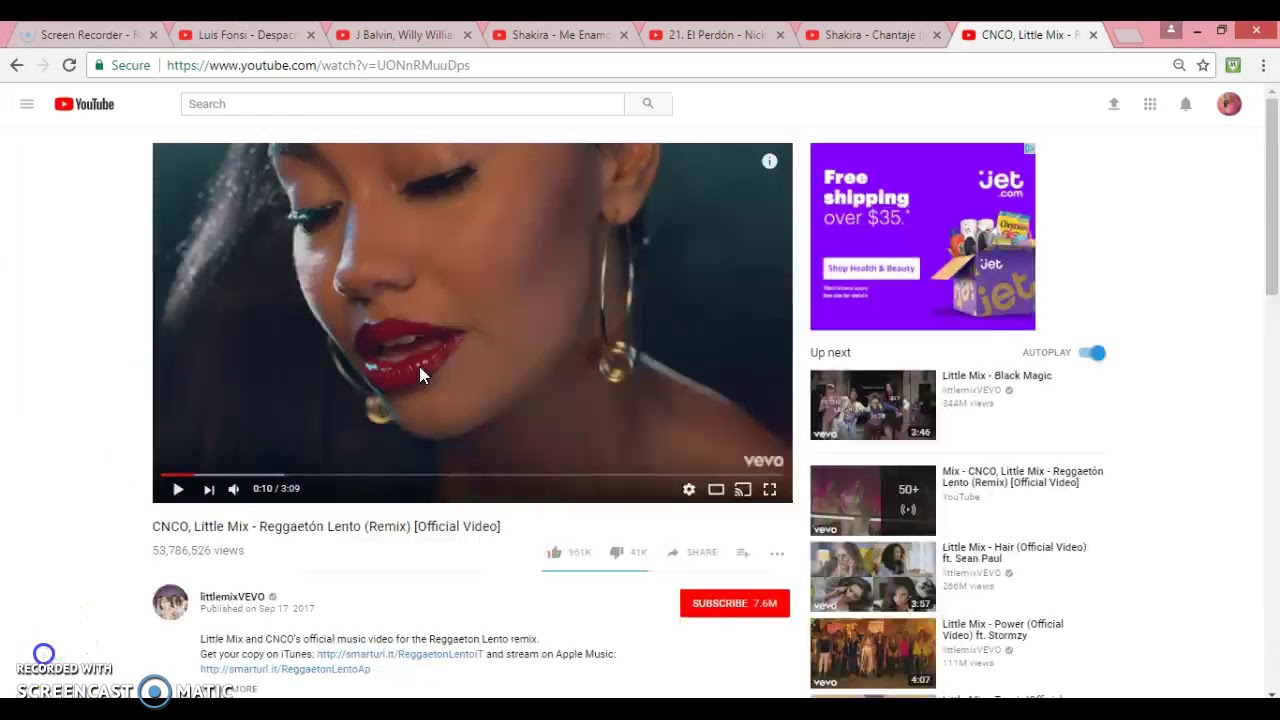This image showcases a browser window displaying YouTube. The current page features the official music video for "Reggaeton Lento (Remix)" by CNCO and Little Mix. The video thumbnail prominently displays a close-up of a woman's face, who appears to have her eyes closed and is facing toward the bottom left. The image is tightly cropped, capturing only her face, part of her neck, and her left shoulder. She is adorned with large circular earrings. The video has garnered approximately 161,000 thumbs up and has amassed 53,786,526 views. On the right-hand side of the screen, there is a "Up Next" section that previews four other video thumbnails.